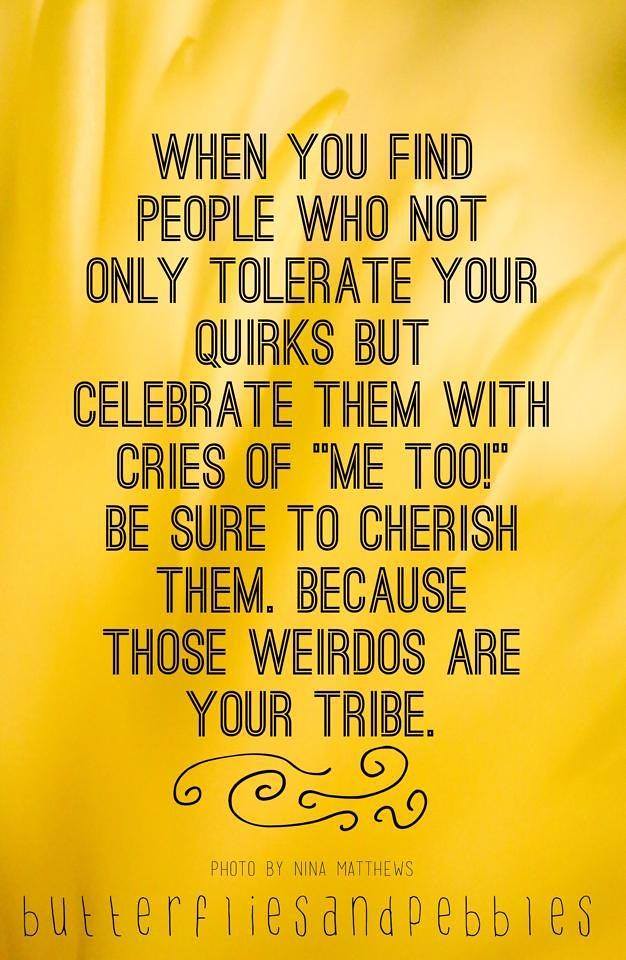This motivational poster, often shared on social media platforms like Facebook, features an uplifting message against a vivid yellow backdrop. The central text, displayed in a friendly, all-caps font with black lettering outlined in white, reads: "When you find people who not only tolerate your quirks but celebrate them with cries of, 'Me too!' be sure to cherish them because those weirdos are your tribe." Beneath this heartwarming quote, four squiggly lines add a whimsical touch. Below these lines, in a smaller font, the credit reads "Photo by Nina Matthews," followed by a larger, slightly faded inscription at the very bottom that says "Butterflies and Pebbles." The background incorporates a blend of various yellows, whites, and golds, enhancing the overall motivational and cheerful vibe of the poster.